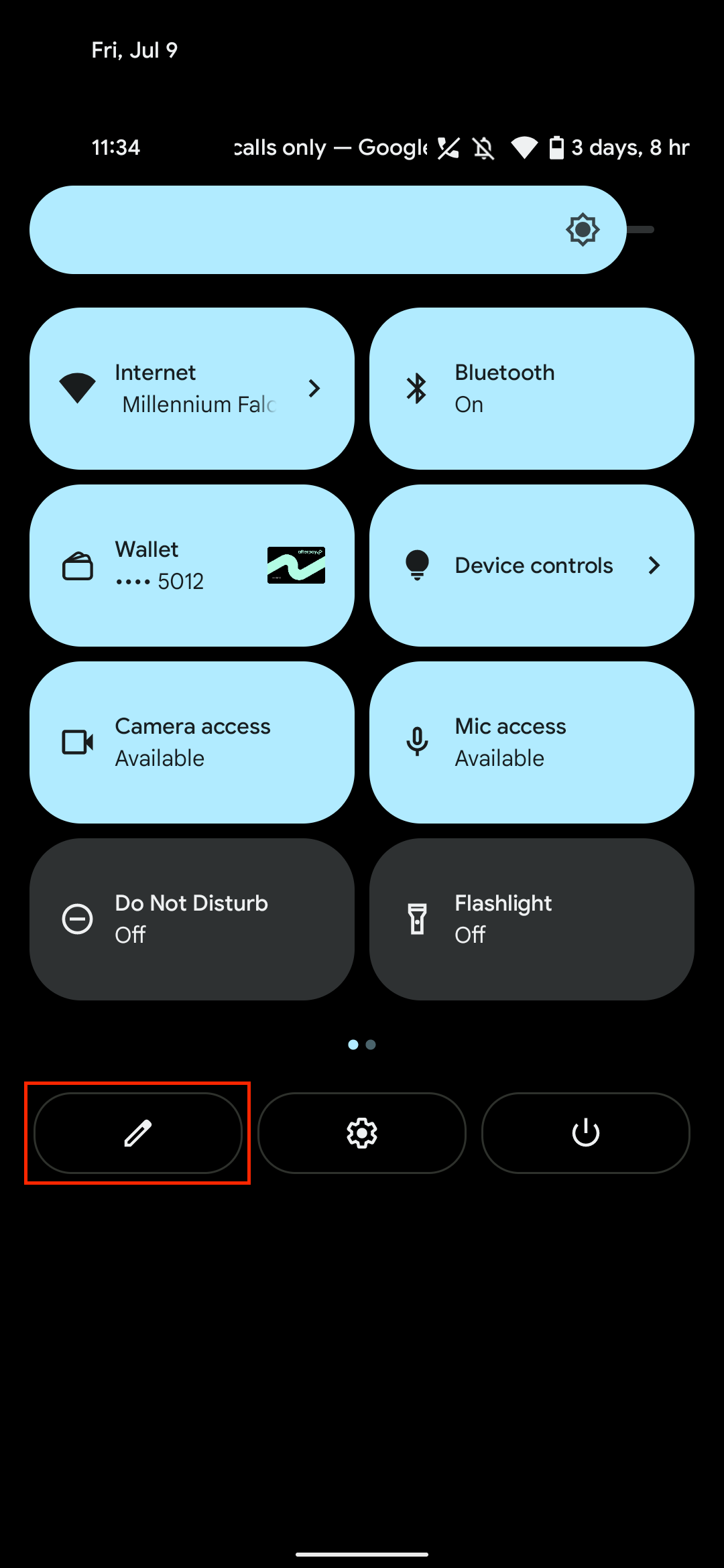This is a screenshot from a mobile phone's interface. The background is pure black. At the very top, in white font, it displays "Friday, July 9th" on the top left corner, and directly below that, "11:34." Further to the right, it states "Calls only - Google," accompanied by a phone handset icon with a slash through it, a bell icon with a slash through it, a fully white Wi-Fi icon, and a battery icon indicating 75% charge along with the text "3 days, 8 hours."

Below this, the dropdown menu typically available on phones is visible, pulled down to show quick settings. At the top of this menu, there is a light blue brightness bar, set almost at its maximum level. 

The next row contains a button labeled "Internet," followed by the text "Millennium Falcon." To the right is a button labeled "Bluetooth on." 

In the subsequent row, on the left, there is a "Wallet..." button with the numbers "5012" and a small credit card icon. To its right is a button for "Device controls."

Finally, the row at the bottom displays two buttons: "Camera access available" and "Mic access available."